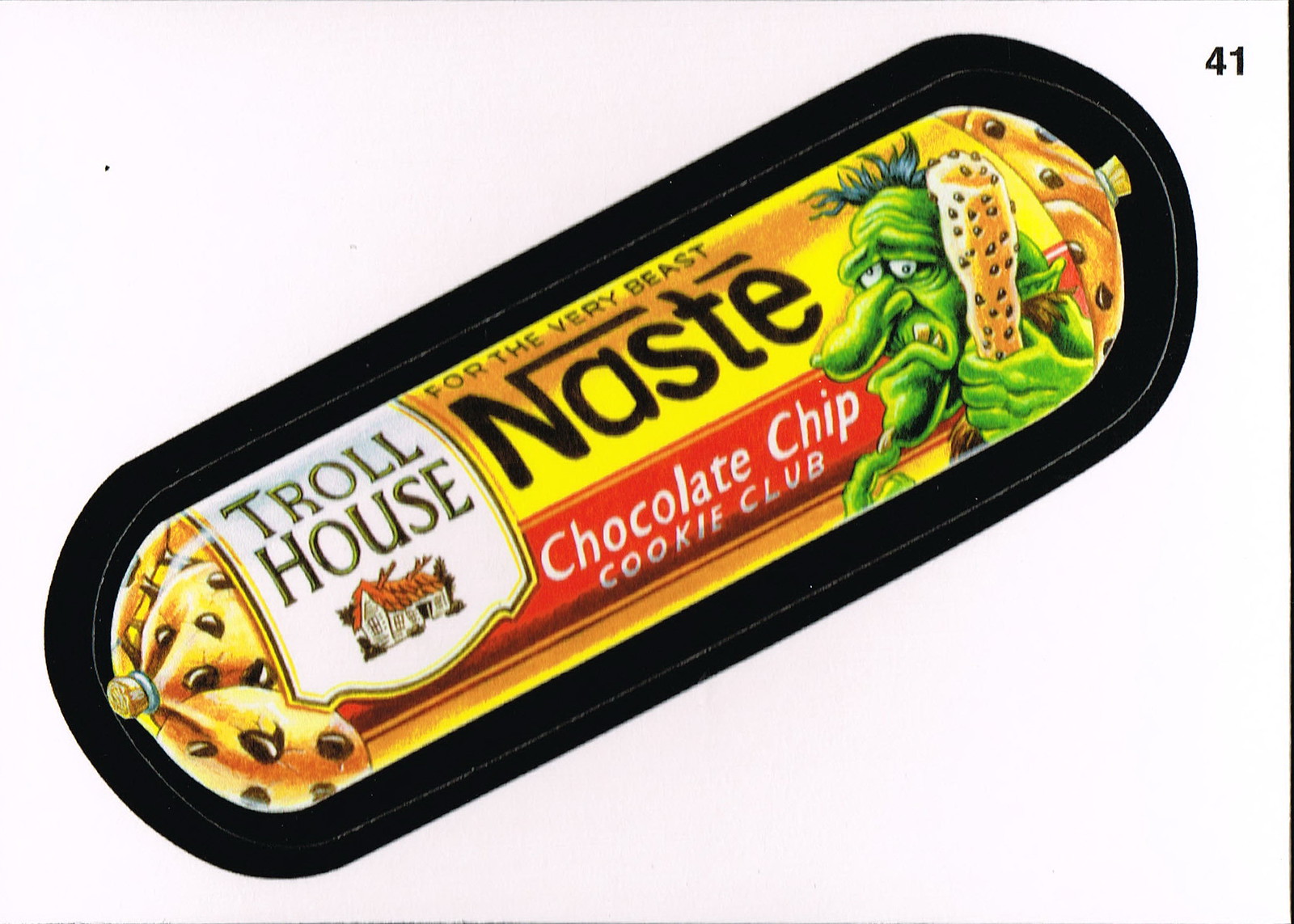This image appears to be a stylized or cartoon-like rendering set against a background resembling a white sheet, which has some darker color noise mimicking shadows. Dominating the right edge is a prominent vertical black line, and in the top-right corner of the image, the number "41" is displayed in black text.

The focal point of the image is a yellow tube with a white label section. This label features the text "Troll House" in dark letters alongside an illustration of a small white house with a red roof. Adjacent to the white section, on the yellow background, the text reads "N.A.S.T.E. For the Very Beast. N.A.S.T.E. Chocolate Chip Cookie Club." Additionally, the tube showcases a whimsical green troll with a long nose, a visible green wart, and a tuft of blue hair atop its head. The troll is depicted holding a club made to resemble cookie dough with chocolate chips.

The tube is humorously designed to parody the well-known brand "Toll House" and is situated within a black tray, emphasizing its playful and illustrative nature.